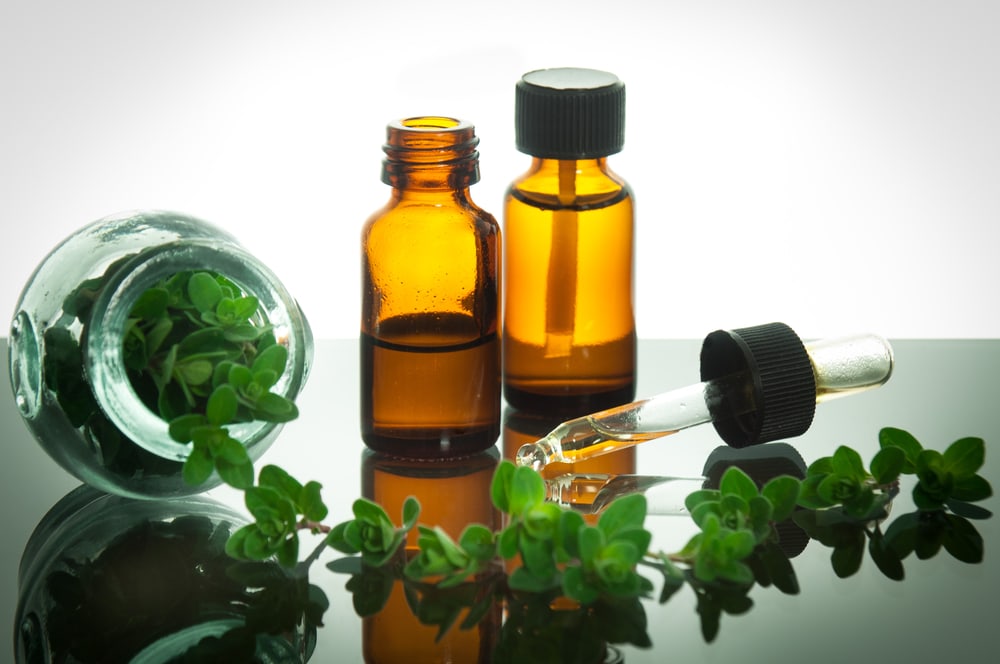The image depicts a photorealistic scene set against a stark white background. At the forefront, there are two amber-colored glass vials containing a clear liquid, reminiscent of medication or chemicals. The vial on the left is open with its black dropper cap lying beside it on the glass tabletop, revealing the vial is only half full. The second vial, positioned to the right, is full and remains sealed with its black cap. Both vials reflect vividly off the glass surface beneath them. Adjacent to the vials, to the left, rests a small glass pot housing a vibrant green vining plant. The plant's vine trails gracefully, intertwining with the dropper cap of the open vial, adding a touch of organic elegance to the otherwise clinical scene. Reflections of the vials, the dropper, and the plant's vine create a mirrored effect on the tabletop, enhancing the image's detailed realism. The composition, with its clear, crisp reflections and minimalistic white background, evokes a sense of calm and precision.